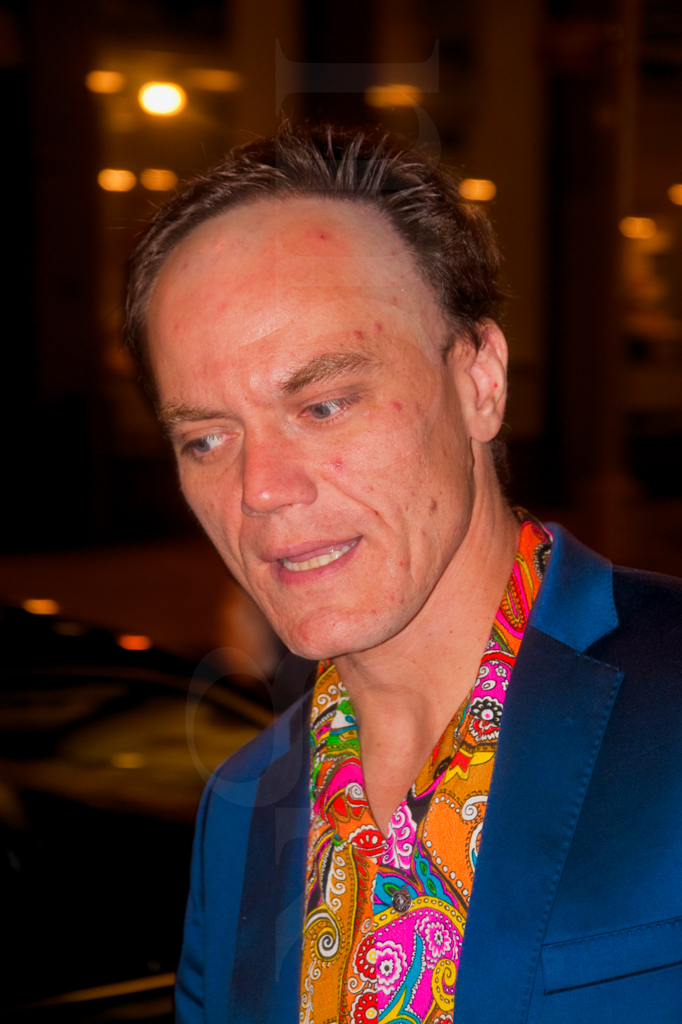This image is a detailed portrait of a white man, possibly in his late 40s, who has pale skin, brown hair slicked back, with parts of his hairline near the front and side shaved away. He is dressed in a vividly colorful, paisley-printed collared shirt that features an array of colors including orange, blue, green, pink, white, red, yellow, and black. Over this shirt, he sports a bright blue, shiny jacket that appears to have a satin or silk-like quality, lending it a slightly reflective sheen. He is positioned towards the bottom right of the image, visible from the chest up, and his head is centered but slightly sticking out, looking downward towards the bottom left. The background is blurry, possibly indicating a street scene at night, with some indistinct lights and a hint of what looks like a black car in the top left corner.